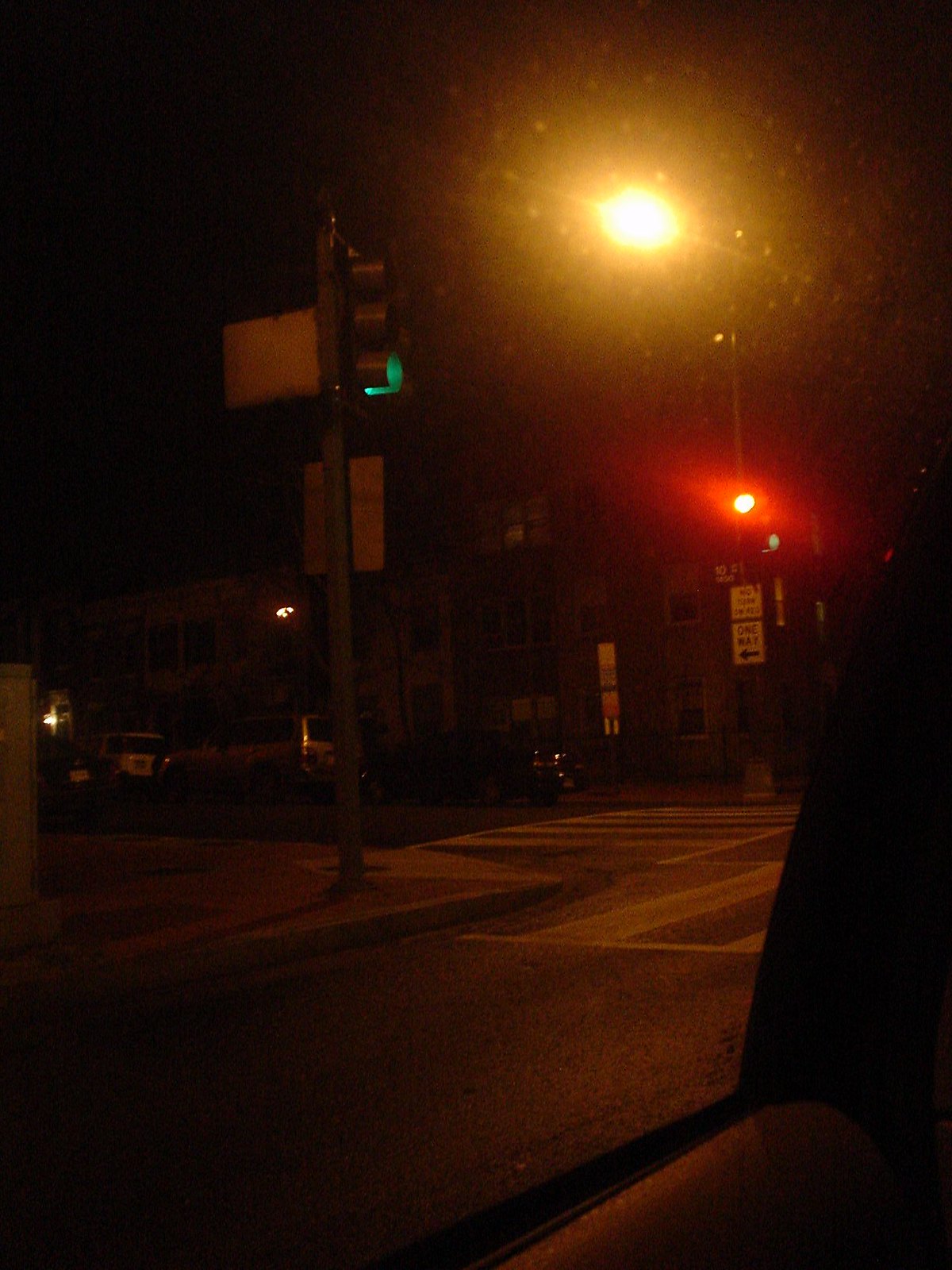A nighttime photograph captures the view from the backseat of a car, looking through the rear passenger window. In the lower right corner of the image, part of the car's door frame is visible. Outside, a street corner can be seen illuminated by a streetlight and a green traffic signal, indicating "go," oriented towards the left side of the photo. In the background, apartment buildings stand under the dim night sky, adding an urban backdrop to the scene.